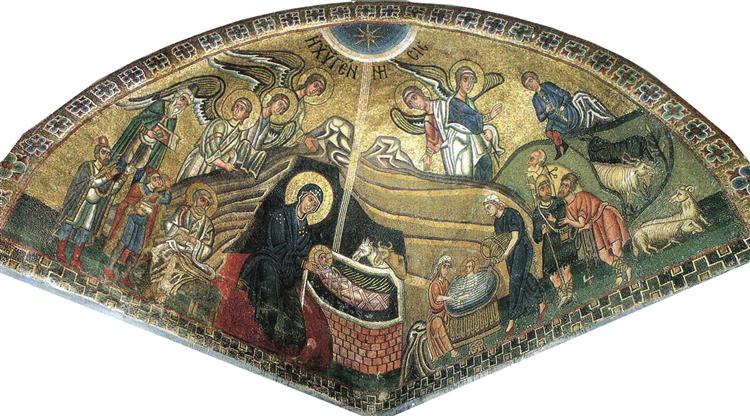This is a detailed color photograph of a section of a religious mosaic or painting, likely adorning the dome of a church. The image predominantly features a golden background with intricate decorative edging. At the center of this Christian scene, a woman dressed in a black robe with a golden halo is seen holding a baby Jesus, who also has a halo and is possibly in a crib.

Surrounding them, the composition includes five or six angels with halos and wings, positioned above and around the central figures. There is a man with a white beard holding a book, accompanied by three smaller figures below him, likely depicting kings or religious figures observing or presenting offerings. Towards the right, the scene extends to display a collection of farm animals, including goats, and several people engaged in conversation. There are also two women depicted carrying another baby in a basket, adding further depth to the narrative of nurturing care.

The image is rich in colors such as gold, green, dark red, and black, and features a range of human emotions and interactions. Additionally, some writing in an unfamiliar script appears at the top of the image in black text. All these elements together create a vivid depiction of a moment from Christian or Catholic mythology, possibly illustrating the nativity or an event from the life of baby Jesus.